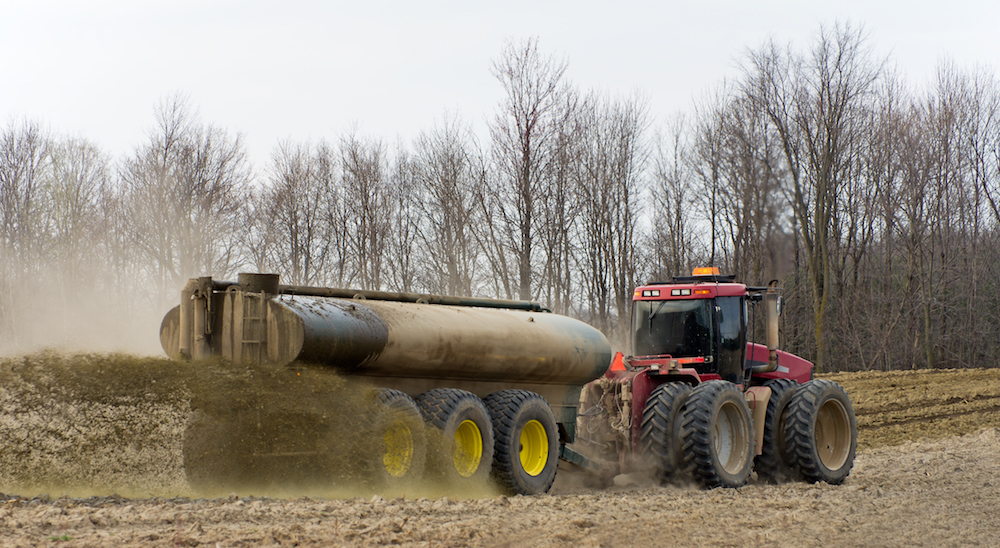The image depicts a robust, red tractor driving from left to right along a muddy dirt road on a farm. The tractor, equipped with eight sturdy black rubber tires—four large wheels in the back and two smaller ones in the front on each side—features a prominent vertical gray exhaust pipe on its hood and an orange safety lamp atop the cab. The cab has blackish but still transparent windows, giving it a muscular and heavy-duty appearance.

Attached to the back of the tractor is a substantial six-wheeled trailer designed to carry a massive canister-like container. Despite some interpretations of the container's contents differing—possibly gas, water, or fertilizer—it's evident from the heavy stream spraying out horizontally that the container is distributing a liquid, likely fertilizer, over a large swath of land. Dirt is visibly kicking up around the vehicle, signaling its active work on the field.

In the background of the photograph, an overcast gray sky looms above a collection of tall, leafless trees, framing this scene of agricultural labors and emphasizing the functional, industrious atmosphere of the farmland.